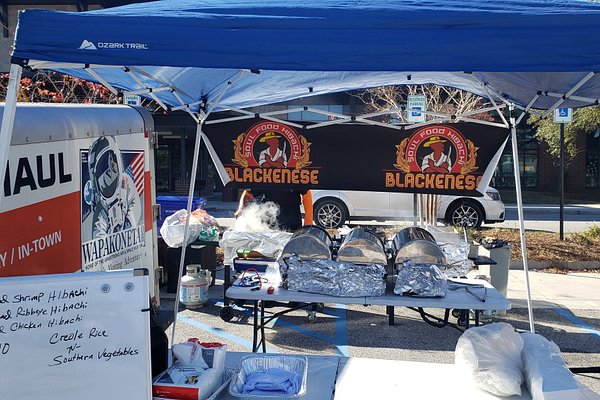The image shows a vibrant setup for a food truck event, likely preparing for a lunch rush. A collapsible canopy awning houses a banquet table laden with food wrapped in tinfoil, beneath which there are several grills and propane tanks for cooking and heating. The banner hanging at the rear of the awning reads "Blackanese Soul Food Hibachi" and features an animated image of an African American man in a straw hat, with arms crossed and holding a knife. To the left of this setup is a small U-Haul trailer with an astronaut painted on its side, and a handwritten display board lists menu items such as shrimp hibachi, ribeye hibachi, chicken hibachi, creole rice, and southern vegetables. Beyond this setup, a white minivan or SUV is partially visible, parked in a wheelchair spot in a parking lot. The scene suggests a bustling outdoor event or festival setting where delicious soul food hibachi is being served.